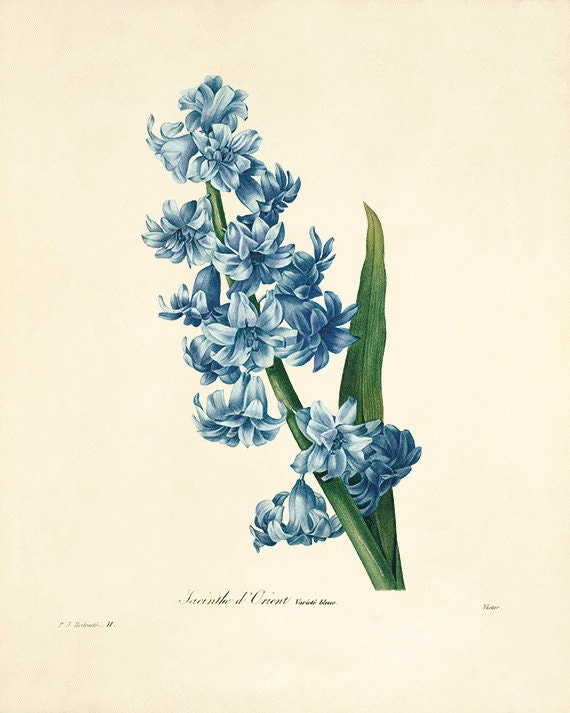The image features a detailed painting of a hyacinth bloom rendered on a peach-colored piece of paper, possibly reminiscent of an old botanical illustration or poster. The plant features a prominent green stem adorned with clusters of delicate, downward-bending blue bell-shaped flowers. A single, large, deep green, elongated leaf with a prominent central vein is visible on the right side of the stem. At the bottom of the image, there is some ornate, illegible text, including the partly visible word "orients." Additionally, there are small writings positioned at the bottom left and right corners of the paper.